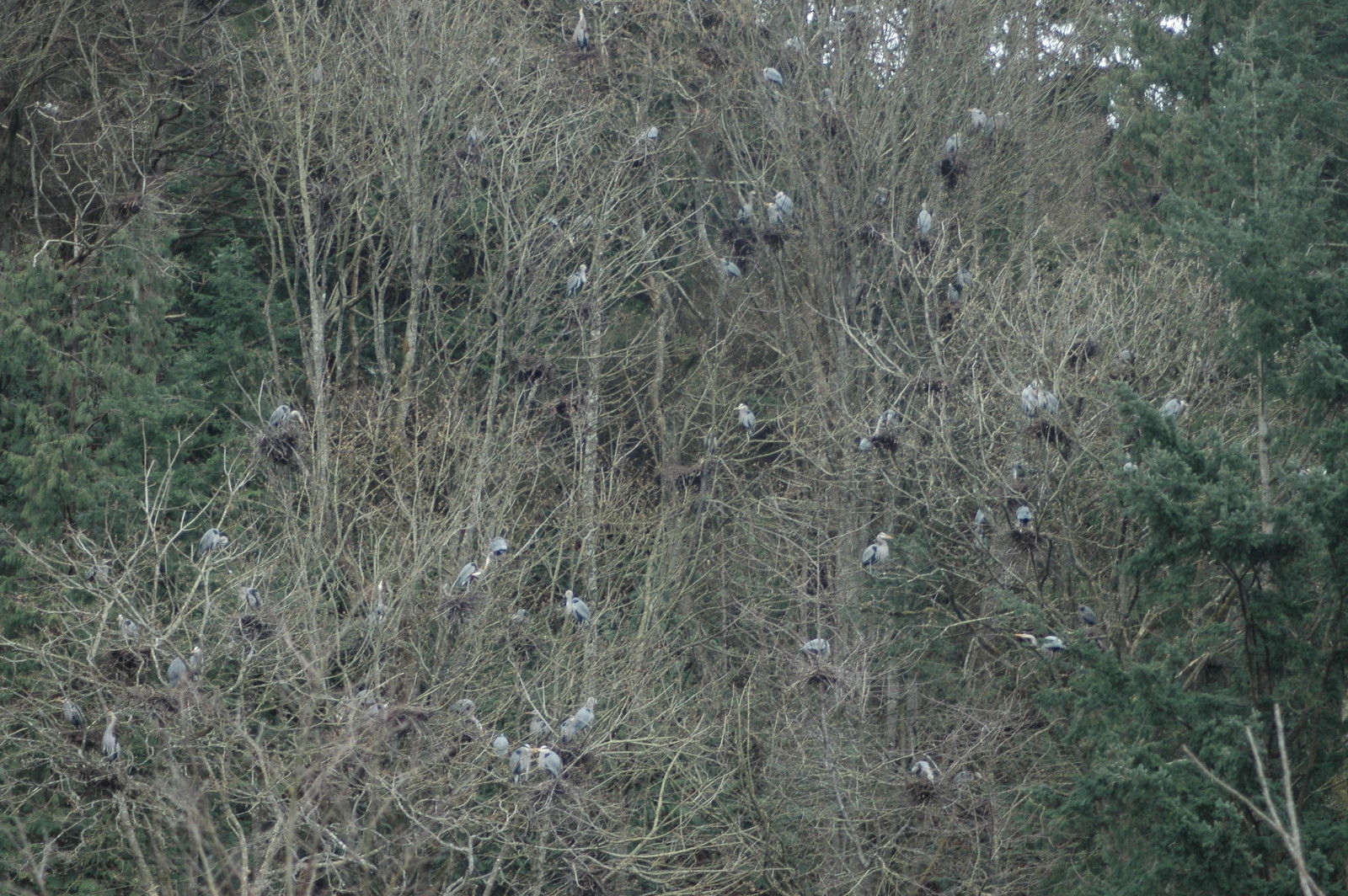The photograph is a darkly lit, color image capturing a large congregation of birds nestled in nearly leafless trees, which suggests a fall setting. The trees, featuring branches that range from light brown to dark brown, are densely populated with these birds, estimated to be between 30 to 40 in number. These birds have white and light gray plumage with distinctive flat markings and a dark blue patch on their shoulders, alongside a lighter yellowish bill. Surrounding these barren trees, which are filled with nests made of intertwined branches, are some evergreen trees, possibly pines. The entire scene, filled with nests and birds scattered throughout, presents a detailed and complex tableau of avian life in a forested area, bathed in muted lighting.